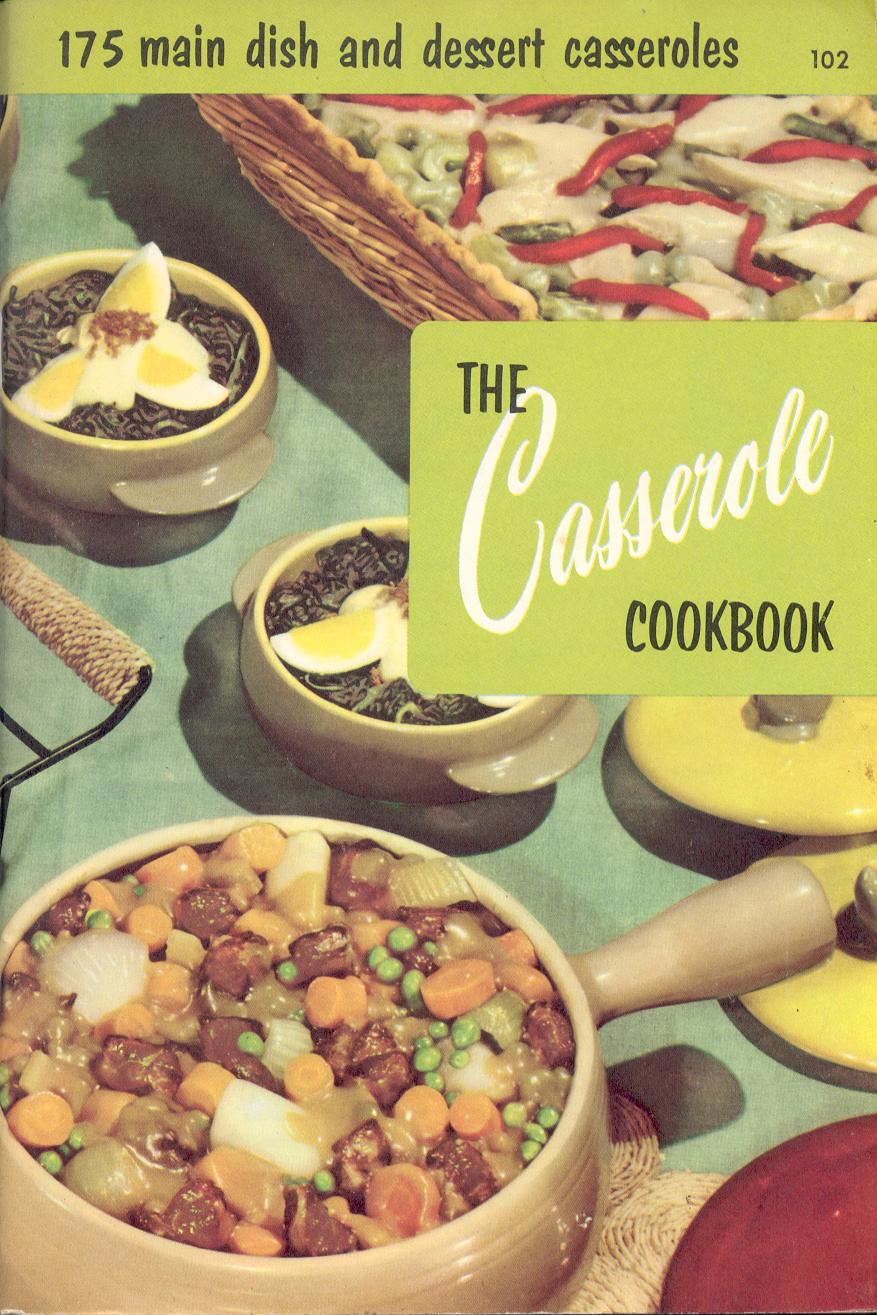The image is a colored photograph of a vintage 1950s-1960s cookbook titled "The Casserole Cookbook." The cover prominently features a rectangular banner at the top with the text "175 Main Dishes and Dessert Casseroles" in black lettering, followed by the number "102." To the right of the banner, the title "The Casserole Cookbook" is displayed, with the word "Casserole" written in large cursive font against a green rectangle, and "Cookbook" in capital black letters below it. The background image on the cover shows a table setting with a green tablecloth, filled with various types of casseroles in ceramic brown pots and dishes. In the foreground on the left, there's a large tan clay pot containing what looks like a beef stew with sliced carrots, peas, potatoes, and ground beef. In the lower right corner, there's another small pot, and in the upper right corner, there is a woven wicker basket holding a casserole with red peppers, onions, and possibly some type of white meat. Another dish in the scene features hard-boiled eggs spread open with some green leafy vegetables, possibly cooked spinach or collard greens, and some kind of sauce. Various pot lids are also scattered throughout the table setting.